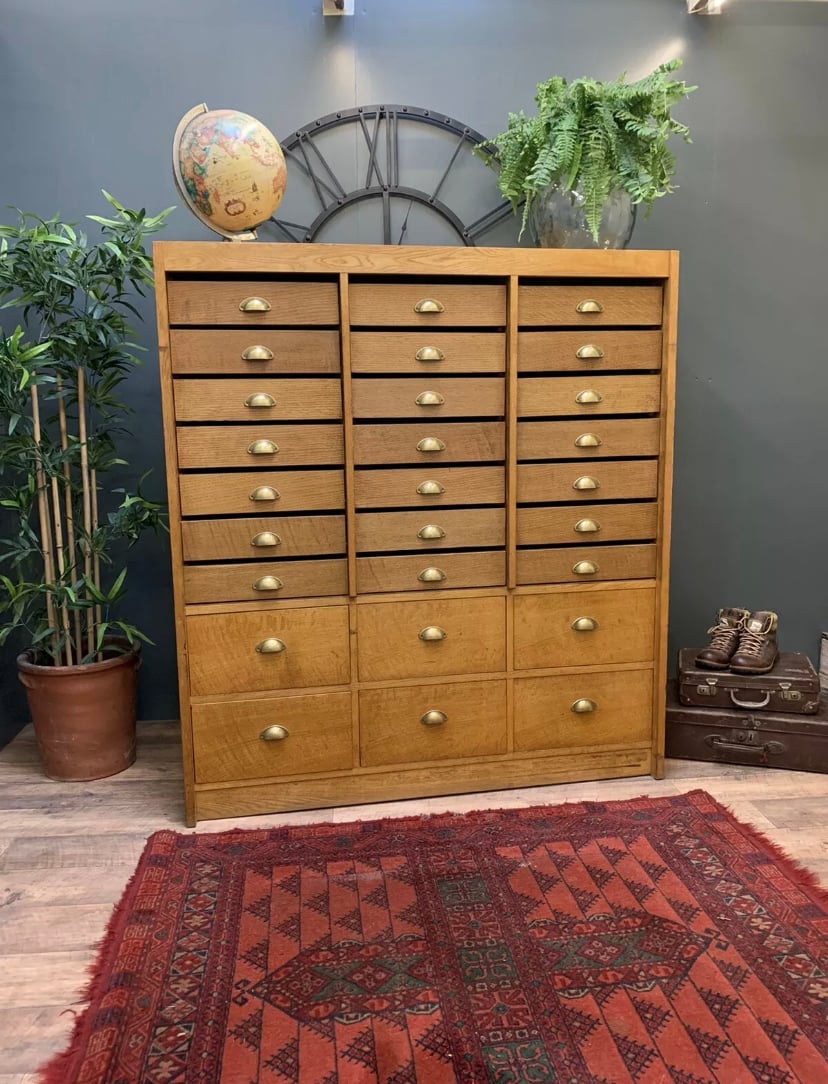The image depicts a vintage wooden dresser, likely made of light wood such as walnut, featuring three columns of drawers. Each column consists of seven shallow drawers, topped with gold or metal handles, followed by two bottom drawers that are about twice the size. Resting on top of the dresser is a vintage globe with a tannish color accented by greens and reds. To the left of the dresser stands a brown pot containing light beige sticks and lush green leaves, including ferns. Adjacent to this, on the right side of the dresser, sits a brown suitcase with two pairs of brown shoes neatly placed atop it. The setting appears to be an indoor room, where a vintage red rug, detailed with patterns in reds and greens, lies in front of the dresser, exhibiting some fraying on its edges.